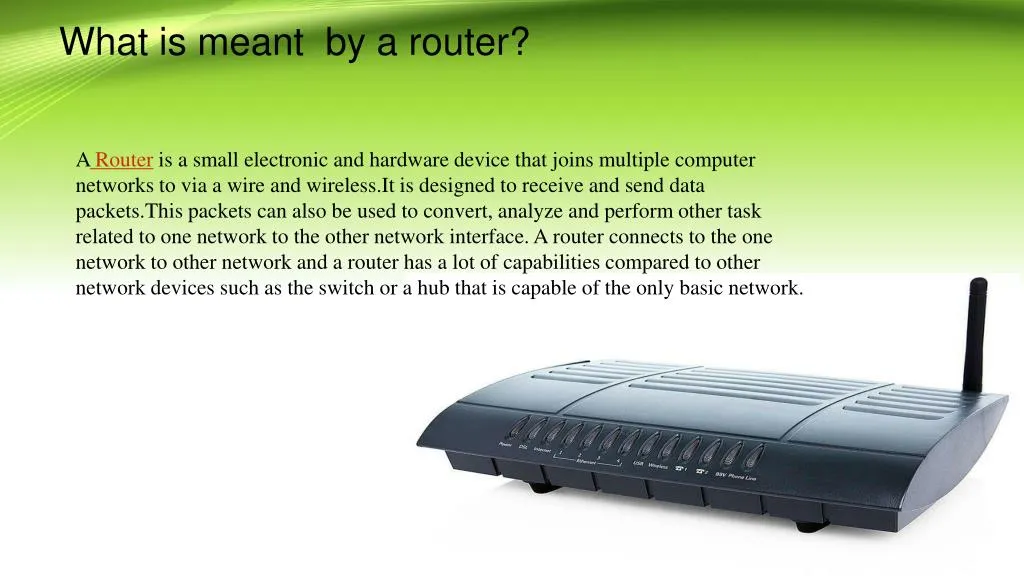The image is an informational PowerPoint slide about routers. The background features a gradient beginning with a dark green at the top, transitioning to light green, and then to white. The slide's title, located at the top in black letters, reads "What is meant by a router?" The subtitle below it, with the word "router" highlighted in red, further states "A router." The primary text describes a router as a small electronic and hardware device that joins multiple computer networks via both wired and wireless connections. It is designed to receive and send data packets that can also be used to convert, analyze, and perform a variety of network interface tasks. Unlike basic network devices such as switches or hubs, routers offer enhanced capabilities and functionalities, allowing one network to connect to another. At the bottom of the slide, there is an image of an older router with a flat, curved-top design. The router has a series of light indicators on the front and a single black antenna on the back right side.